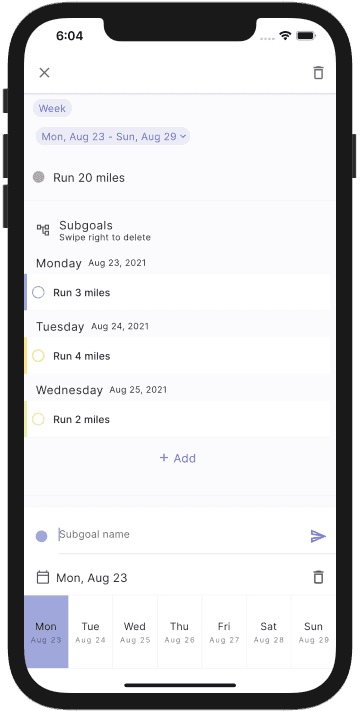The image depicted is a detailed screenshot of a smartphone displaying a digital workout plan. The top section of the screen shows typical elements of a phone interface: an Apple icon in the top left, the time "6:04," and indicators for full signal bars and a fully charged battery on the right. No cell service is connected.

Just beneath this, there is an 'X' icon for closing the menu. Adjacent to it on the right, there appears to be a trash can-like symbol, though its exact nature is unclear.

The main portion of the screen displays a fitness schedule for the week of Monday, August 23rd to Sunday, August 29th. The selected week is highlighted. Below this section, a gray checkmark icon precedes the target “Run 20 miles”, outlining the weekly goal. The list further breaks down daily objectives:

- **Monday, August 23rd, 2021:** Run 3 miles (unchecked)
- **Tuesday, August 24th, 2021:** Run 4 miles
- **Wednesday, August 25th, 2021:** Run 2 miles

At the bottom of Wednesday's task, there's an option to add more goals, indicated by a "+" add button and a field to input a sub-goal name.

The interface's background is predominantly white, with the navigation options for each day of the week from Monday to Sunday listed at the bottom of the screen. This allows users to navigate to specific days and view or update their planned activities.